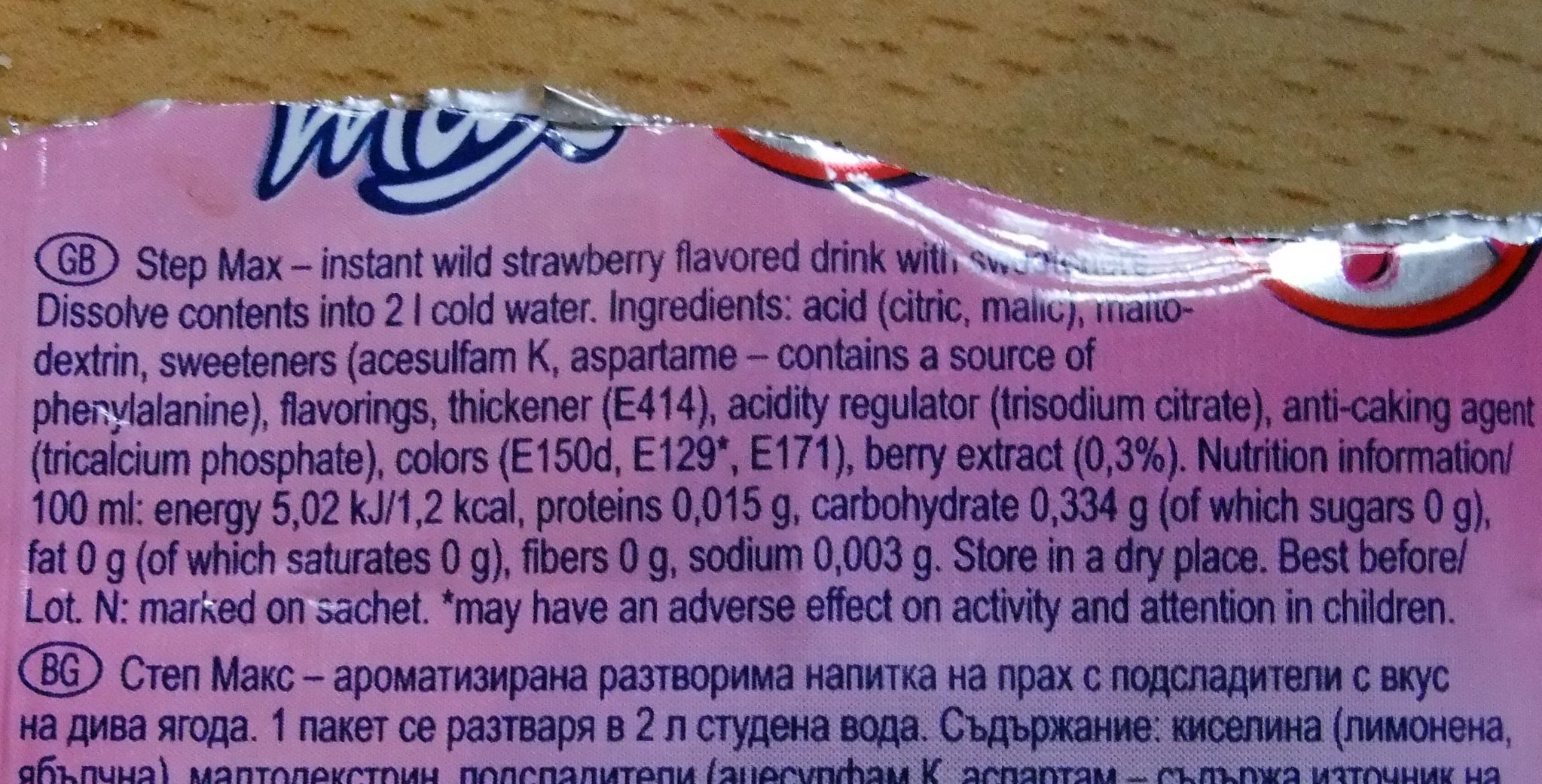The image depicts a torn piece of a nutrition label that appears to belong to a flavored drink product. The fragment rests on a wood-grain surface, likely a table, with only the top third of the label visible against the background. The label is clearly of Russian origin, as evidenced by the Cyrillic lettering at the bottom.

The top portion of the label reads "Stepmax Instant Wild Strawberry Flavored Drink," indicating that the product is a strawberry-flavored instant beverage mix. Instructions suggest dissolving the contents into two liters of cold water. The label also provides detailed nutrition information and storage instructions, emphasizing the need to keep the product in a dry place. Additionally, it includes a warning that the drink may have adverse effects on the activity and attention of children, hinting at its stimulating properties similar to those of energy drinks like Red Bull.

The ingredient list mentions components such as maltodextrin, acids, sweeteners, flavorings, anti-caking agents, and colorings, identifying the product as a powdered mix intended to create a strawberry-flavored drink.